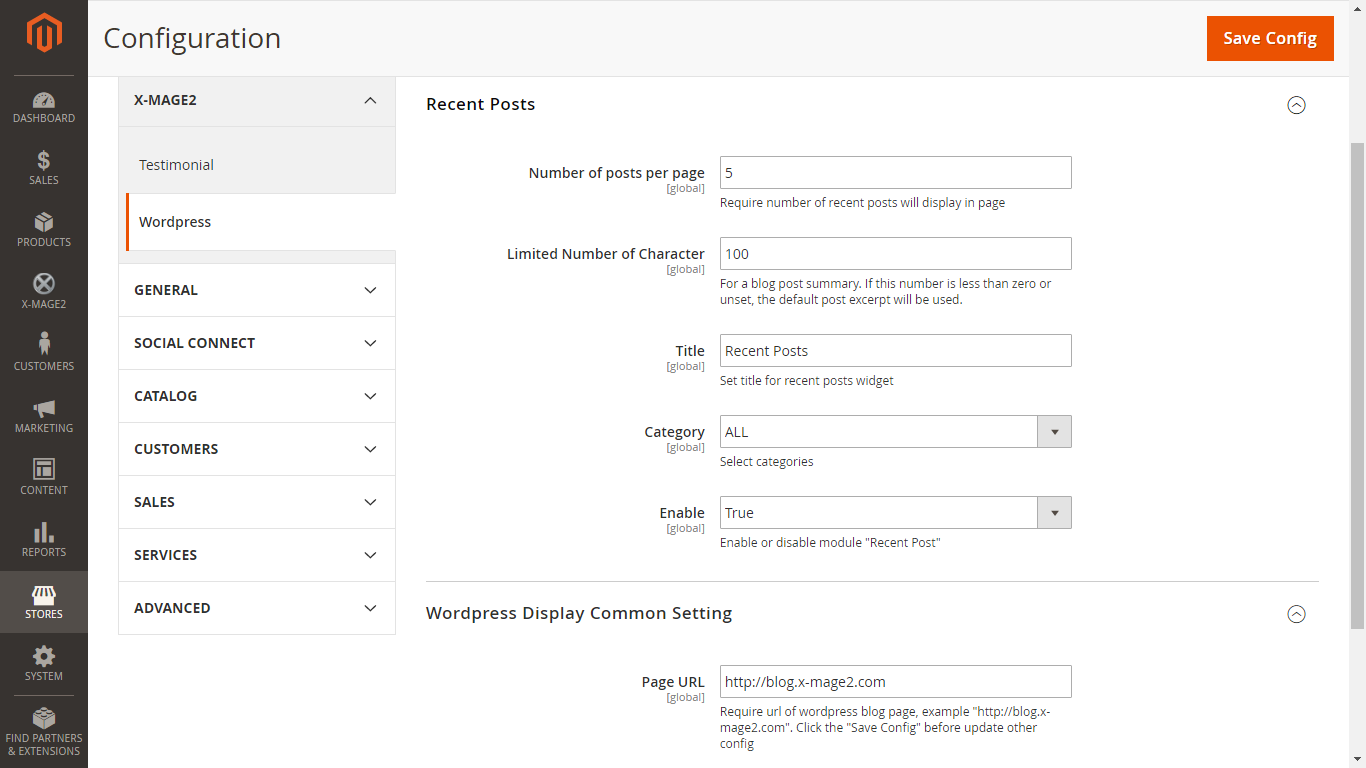In the provided image, the focus is on the configuration settings screen for a system interface. The background is black, and on the left side, a vertical list of options is presented using icons. These options, listed from top to bottom, include: Dashboard, Sales, Products, X-Mage, Customers, Marketing, Content, Reports, Stores, and System. At the bottom of the list, there are additional options labeled "Find Partners" and "Extension." 

Currently, the "Stores" option is highlighted, indicating its selection, and at the top of the interface, the title "Configuration" is displayed. On the top right of the screen, there is a prominent, orange "Save Config" button.

On the right side of the screen, detailed configuration settings are shown under various drop-down menus such as X-Mage 2, Testimonials, WordPress, General, Social Content, Catalog, Customers, Sales, Services, and Advanced. In this instance, the "WordPress" section is expanded and highlighted, revealing more specific settings under the "X-Mage 2" header within WordPress.

In the "WordPress" settings area, the following configuration options are listed:

- **Recent Posts**: Specifies the number of posts to display per page, currently set to 5.
- **Limited Number of Characters**: Defines the maximum character limit for a blog post summary, set to 800. If the number is less than zero or uncertain, a default excerpt will be used.
- **Title**: The title for the recent posts feature, specified as "Recent Post."
- **Subtitle for a Sales Point Widget**: This field is addressed but content is unclear.
- **Category**: Set to include all sales categories.
- **Enable/Disable Module**: The option to enable or disable the recent posts module.

At the bottom of the WordPress settings section, there is a display for common settings and the URL for the WordPress blog page, along with a template example. Users are instructed to click the "Save Config" button before making any updates or adding new configurations.